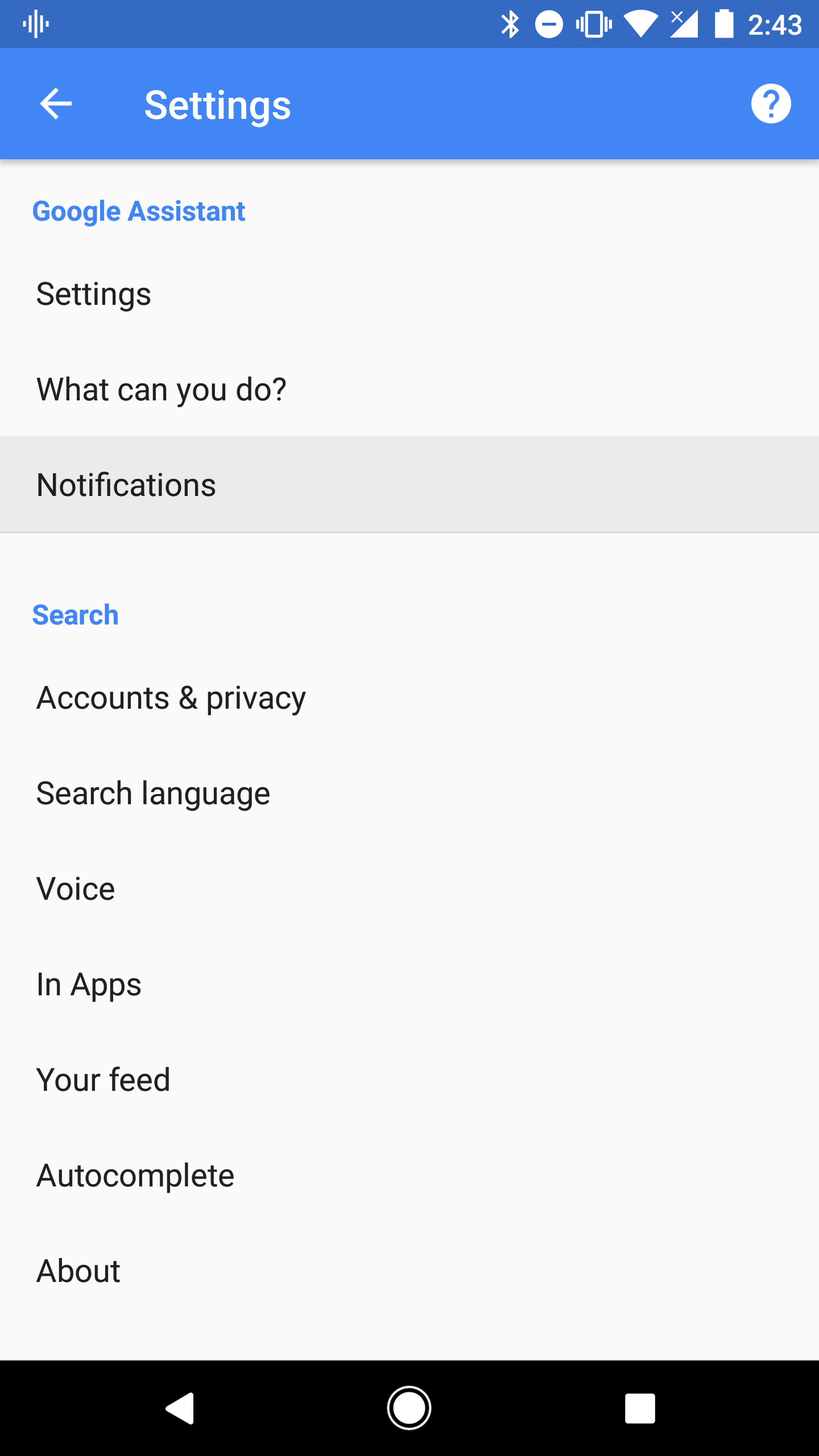The image illustrates an application settings page, prominently displaying the title "Settings" in white against a blue header. To the left of the title is a back arrow icon, while a question mark icon enclosed in a white circle for help is situated to the right.

Beneath the header, the background shifts to white, with "Google Assistant" written in blue as a subheading. Underneath "Google Assistant," there are three options: "Settings," "What can you do?" and "Notification." The "Notification" option is highlighted with a grey outline, indicating it is currently selected.

Further down the page, another blue subheading titled "Search" appears. Below this subheading, a variety of settings are listed in black text on a light grey background. These options include:

- Account and Privacy
- Search Language
- Voice
- In-Apps
- Your Feed
- Auto-Complete
- About

The text in blue acts as subheadings, categorizing the different settings for easy navigation. The detailed layout of the settings page ensures that users can efficiently manage their preferences within the app.